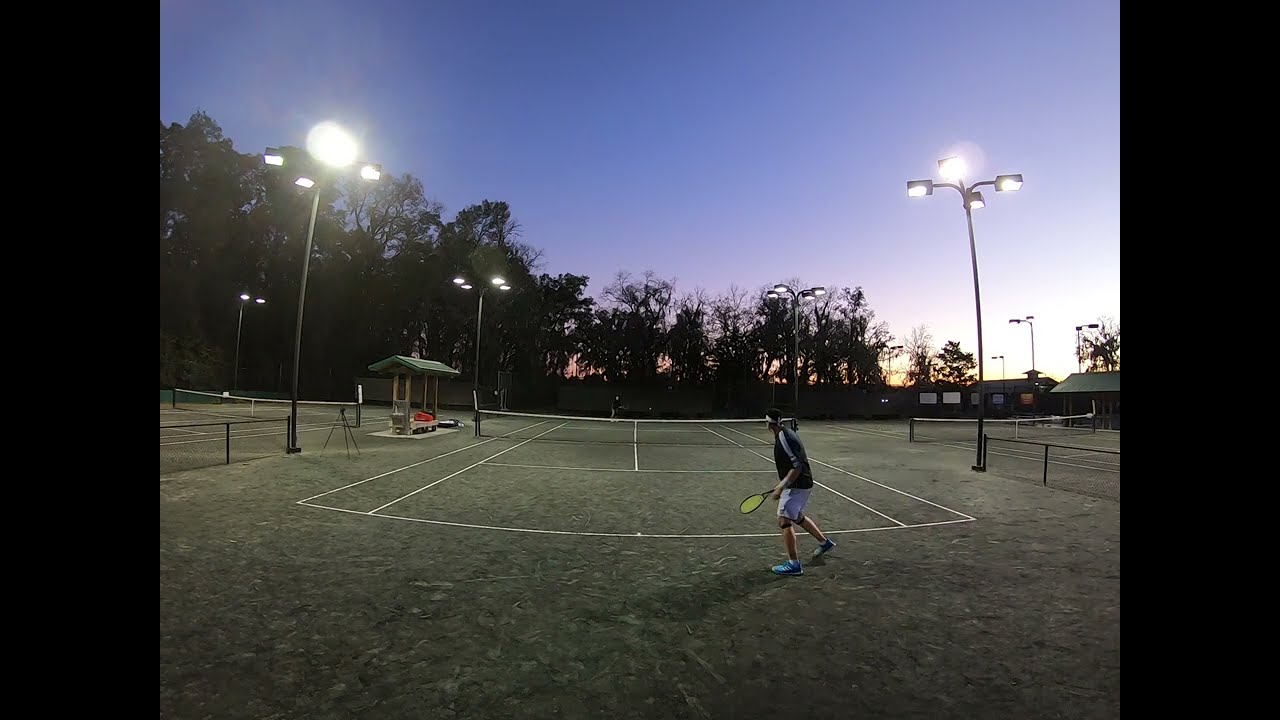This horizontal rectangular image, framed with thick black borders on either side, depicts a vibrant scene of a city park tennis court at twilight. The court is illuminated by multiple street lights positioned along either side, creating a play of shadows and light. The sky transitions from the soft hues of sunset—a gradient from light blue and yellow on the right side to a darker blue on the left—indicating that the sun is either rising or setting. In the foreground, yet at some distance, a tennis player clad in white shorts, a blue top, and a bandana, is captured mid-motion as he runs to hit an unseen ball. The court, with its characteristic white lines and possibly clay surface evident from the footprints, stretches out to another player at the opposite end, though partially obscured by distance. Flanking the court are additional courts and structures, including a covered bench area for seating and a few rest booths. Behind this dynamic scene, a line of trees forms a natural barrier, silhouetted against the gradually darkening sky. The scene is calm yet charged with the energy of the match, encapsulating a fleeting moment in an everyday urban park setting.